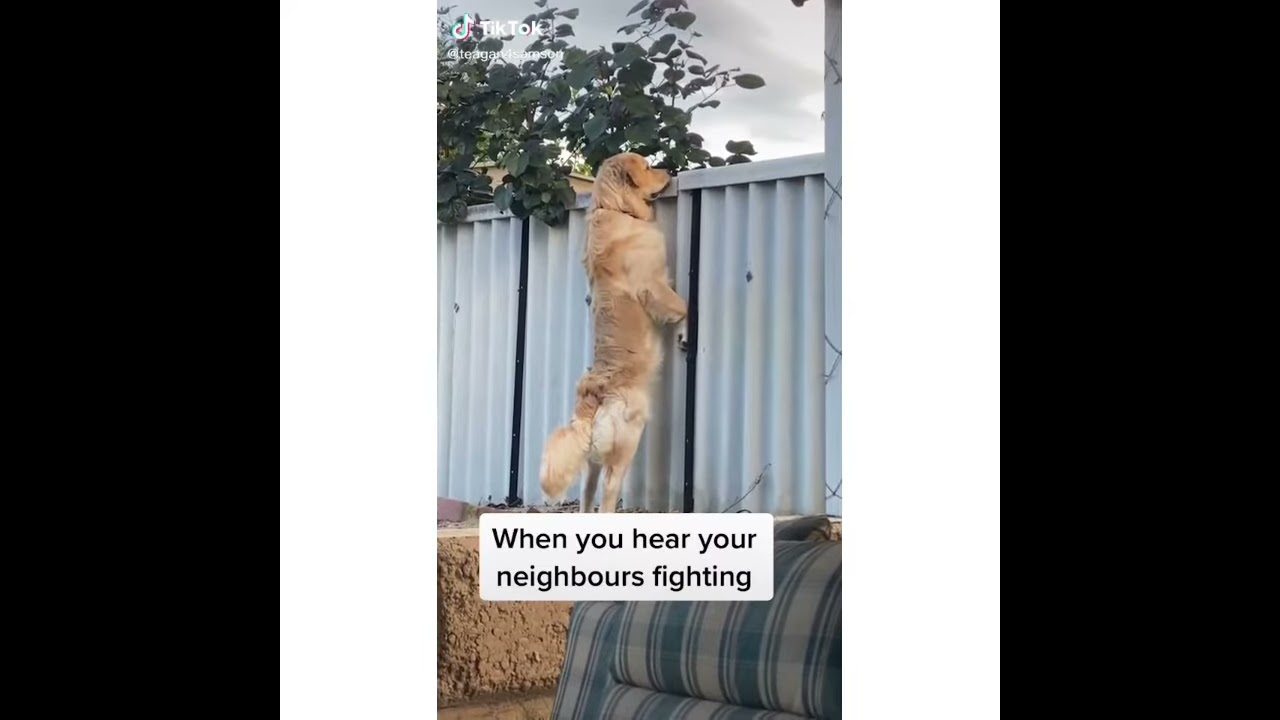This is a TikTok screenshot depicting an outdoor scene featuring a tan-colored, fluffy golden retriever or Labrador retriever mix. The dog stands on its hind legs, peeking over a metal corrugated fence that appears silverish or white. The photograph is set against an industrial backdrop with green leaves from a tree visible behind the fence and a bit of sky with white clouds. In the foreground, there's an incongruous sofa seat, suggesting a possibly cluttered or junkyard-like setting. The TikTok logo is present in the upper left corner, and the image is letterboxed with vertical black and white strips on either side. A white caption at the bottom of the image reads, "When you hear your neighbors fighting," adding a humorous context to the dog's curious stance.